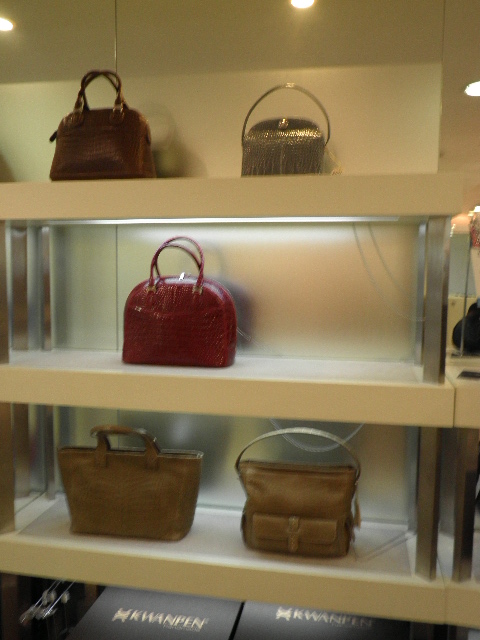This slightly blurry and poorly lit color snapshot captures a minimalist and luxurious store display of handbags. The display features three levels of matte gold-colored or beige-colored shelves, each illuminated with under-shelf fluorescent lights. The bottom shelf holds two tan, large leather handbags with handles standing straight up, one with a strap around the front. Underneath the shelves, there are some black cardboard boxes with gold lettering, though the text is not legible due to the blurriness and possible language barrier. The middle shelf displays a single, distinctive red half-oval leather purse with arched handles positioned on the left. The top shelf showcases a brown leather purse next to a shiny, metallic-looking silver purse. The entire scene exudes a luxurious yet minimalist vibe, with stark shelving and minimal decoration.